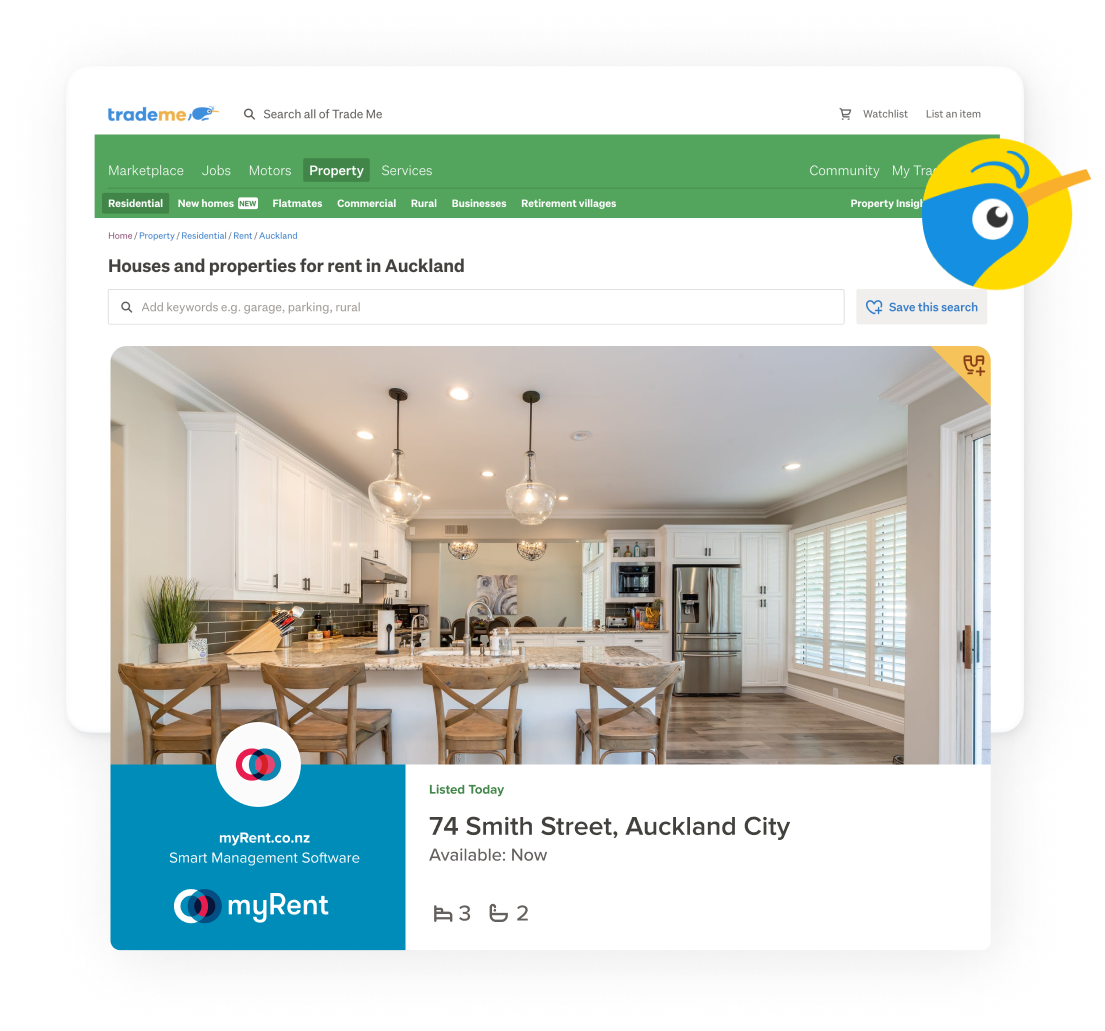The screenshot reveals a section of the Trade Me website, where the company's name is distinctly visible in the top left corner against a white background. The name "Trade Me" is written as one word in lowercase letters, with "trade" in blue and "me" in yellow. Below this, a green header displays menu items in white text, including "marketplace", "jobs", "property", and "services."

Further down, the background shifts back to white, and a bold heading on the left announces "Houses and properties for rent in Auckland, New Zealand." A prominently placed, expansive search box spans the width of the webpage, inviting users to input their criteria.

Beneath this search feature is an enticing photograph of a rental property. The image showcases a sleek, modern apartment with an open floor plan. The vantage point is from the kitchen, offering a clear view of a stylish breakfast bar equipped with four bar stools. To the right, a beautiful hardwood floor stretches out, leading to almost floor-to-ceiling windows that bathe the room in natural light. A gleaming, stainless steel French door refrigerator is elegantly built into the cabinetry.

The left side of the image highlights the kitchen area, featuring pristine white cabinetry and countertops, emphasizing the clean, contemporary design. Below this descriptive section, the listing details are provided, indicating the property was "listed today" and is located at "74 Smith Street, Auckland City," and is "available now."